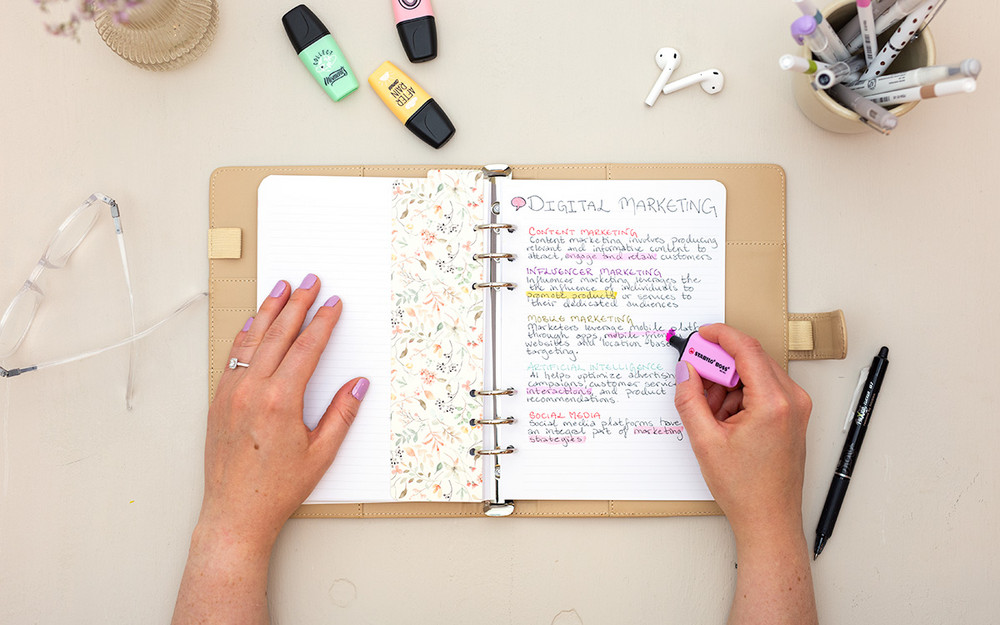In the center of the image, a woman is highlighting a paper titled "Digital Marketing" with a pink highlighter. Her left hand, adorned with a diamond ring and pink nail polish, holds down the page on the left side of a beige leather journal, while her right hand manages the highlighter. The journal is organized and color-coded with various flowery pages and paragraphs in red, purple, yellow, pink, and blue. Surrounding the journal on a tan table are several office supplies: to the right, a black pen, and a white cup filled with pens in colors such as purple, teal, pink, tan, green, and black, along with a pair of AirPods. Above the journal, there are additional highlighters in mint green, yellow, and coral. To the left, there is a pair of clear-rimmed glasses and a small clear glass vase with some blurry flowers. The workspace is meticulously arranged, providing an efficient and aesthetically pleasing setting for her task.